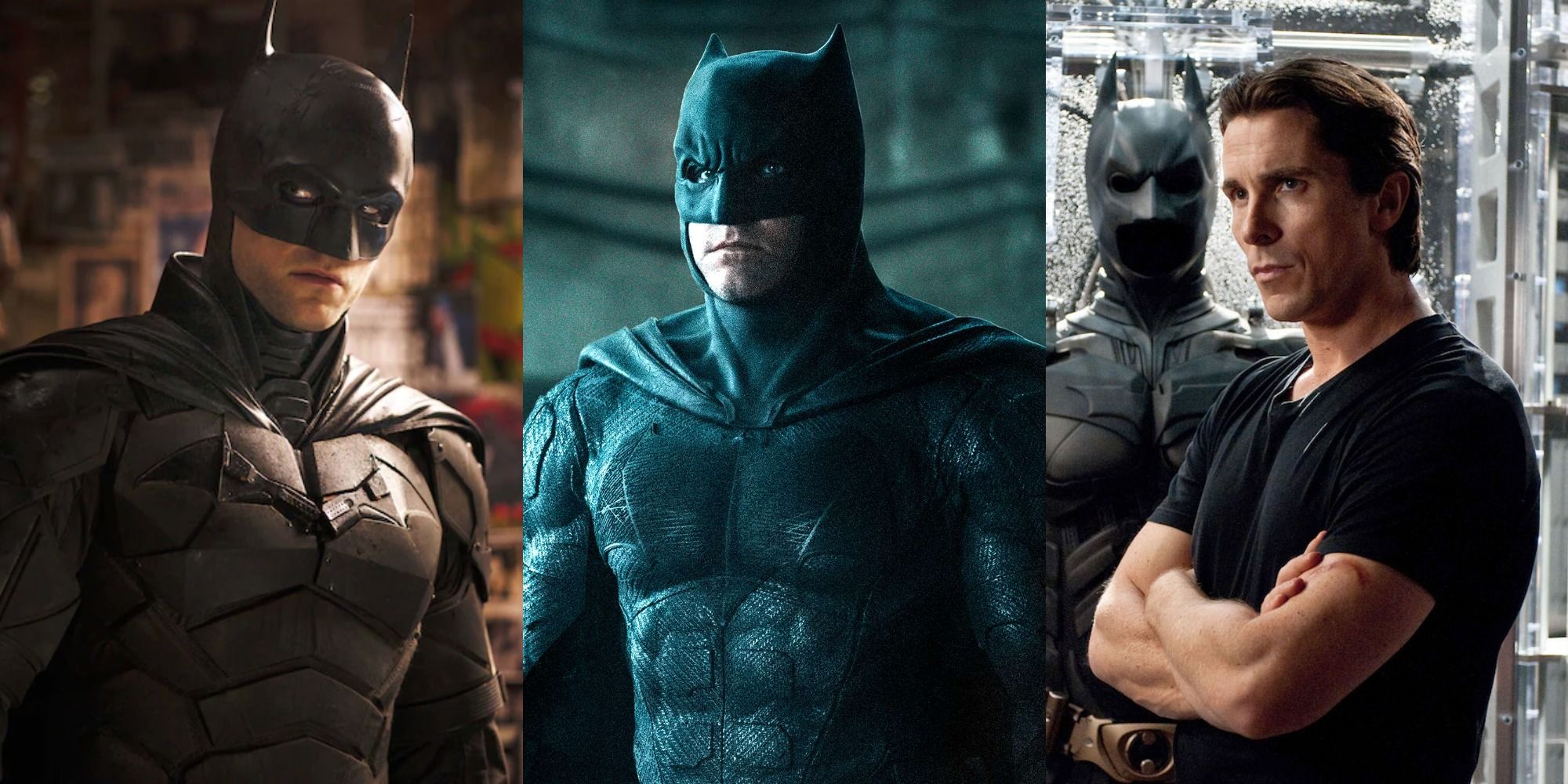The image consists of three distinct photographs of Batman, likely featuring the actors from recent Batman movies, with Robert Pattinson possibly as one of them. The photograph on the left showcases Batman in a full black suit with a prominent bat logo on his chest, set against a blurry background filled with connected newspapers, giving a gritty, investigative ambiance. In the middle, Batman appears particularly buff, also clad in a full black costume, and is set against a rusted, cave-like backdrop, adding to the rugged atmosphere. Finally, the photograph on the right focuses on the actor portraying Batman out of costume, dressed in a simple black t-shirt with a stern expression and arms crossed, looking off to the left; behind him, the Batman suit is slightly visible, emphasizing the duality of his character. These images together underscore the enigmatic and intense nature of Batman through different scenes and settings.